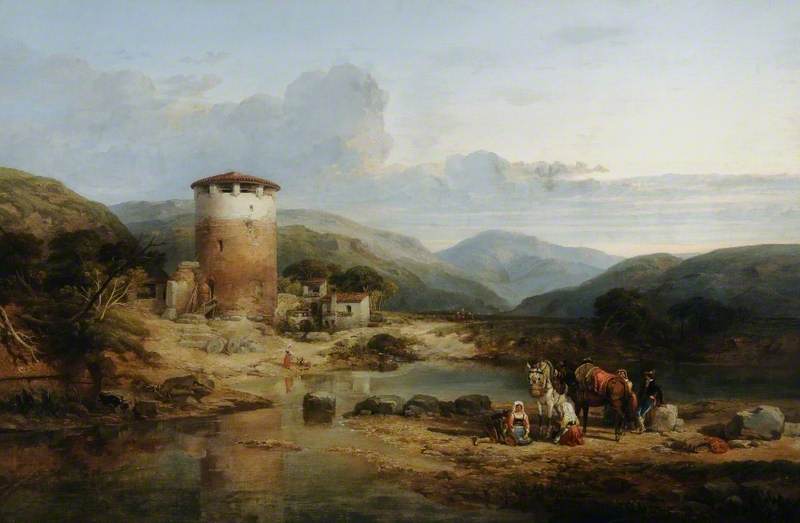This detailed painting captures an outdoor scene characterized by a blue sky adorned with layers of clouds. The background showcases soft, rolling green hills that create a serene setting. In the mid-ground, a small blue pond or lake is divided by a stream with strategically placed boulders, creating a sense of depth and natural flow. To the left, a tall, cylindrical stone tower with a rounded hat-like roof stands prominently, accompanied by white buildings with red tiled roofs nearby. 

In the bottom right of the image, the ground appears earthy and somewhat muddy, likely from the water that runs through it. This area features two horses, a gray and a bay horse, accompanied by four figures. Two women are kneeling on the dirt ground, dressed in long skirts, blouses, and white hoods or head coverings, likely resting. The two other figures are partially obscured behind the bay horse, with one man noticeable leaning against a boulder, contributing to the scene's pastoral and tranquil quality.

Throughout the image, trees in full leaf are dispersed, adding splashes of green to the scene. The distant background reveals additional structures, a stone bridge, and the expanse of mountains under a vast sky filled with clouds. The overall color palette is earthy, enhancing the natural and calm atmosphere of this beautifully rendered older style painting.